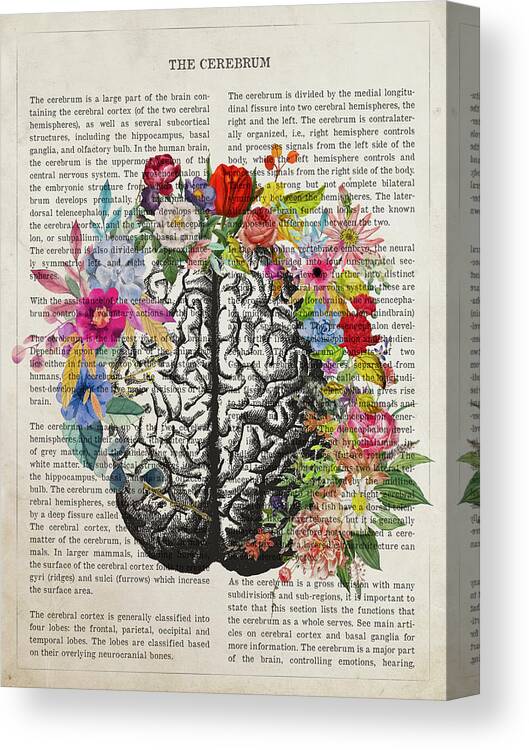The image features a three-dimensional, artistic composition that resembles a torn page from a book or possibly the back cover of a book. It has a grayish background with a thin black border. The title "The Cerebrum" is displayed prominently at the top in bold, all-caps typeface. Below the title, the page is filled with two columns of small Times New Roman font text. 

At the center of the page is a detailed, black-and-white top view of a human brain, which overlays parts of the text. Surrounding the brain is an array of vibrant, colorful flowers, including roses, lilies, and lilacs, in hues of red, pink, purple, blue, orange, and yellow. Green leaves intermingle with the flowers, framing the brain and adding to the ornate, floral display. The combination of the black and white brain with the vivid flowers creates a striking contrast, making the floral details pop against the muted textual background. The angle of the image suggests a slight three-dimensional effect, giving it depth and making it appear as if the flowers are emerging from the brain.